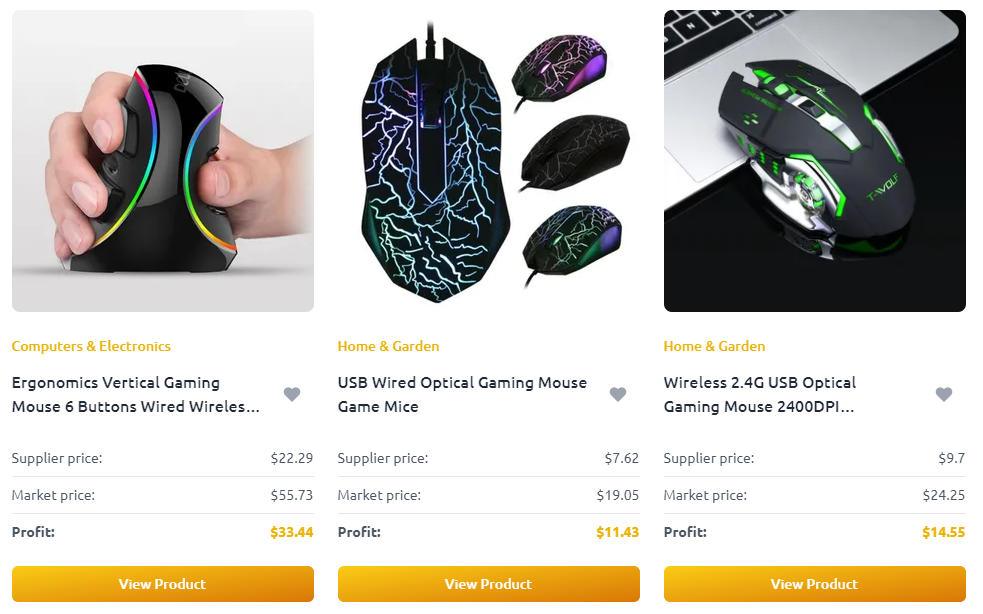On a shopping website, there are three product listings for computer mice. Each listing is displayed vertically in a rectangular format, with the following layout:

1. **Product Thumbnail**: Positioned at the top of each listing, showcasing an image of the respective mouse.
2. **Category Label**: Located just below the thumbnail on the left side, oddly labeled as "Home and Garden" instead of "Computers and Electronics."
3. **Product Description**: Situated beneath the category label on the left side, briefly describing the mouse.
4. **Save Icon**: A heart icon appears to the right of the product description, allowing users to save the item to their wishlist.
5. **Pricing Information**: To the right of the heart icon, three values are provided - the supplier price, the market price, and the potential profit.
6. **Call-to-Action Button**: An orange "View Product" button is located at the bottom of each listing.

The first listing features a USB wired mouse under the miscategorized label "Home and Garden." Similarly, the second and third listings also fall under the same incorrect label, despite showcasing an optical wireless gaming mouse. This layout repeats across all three listings, highlighting an inconsistency between the category label and the actual product type.